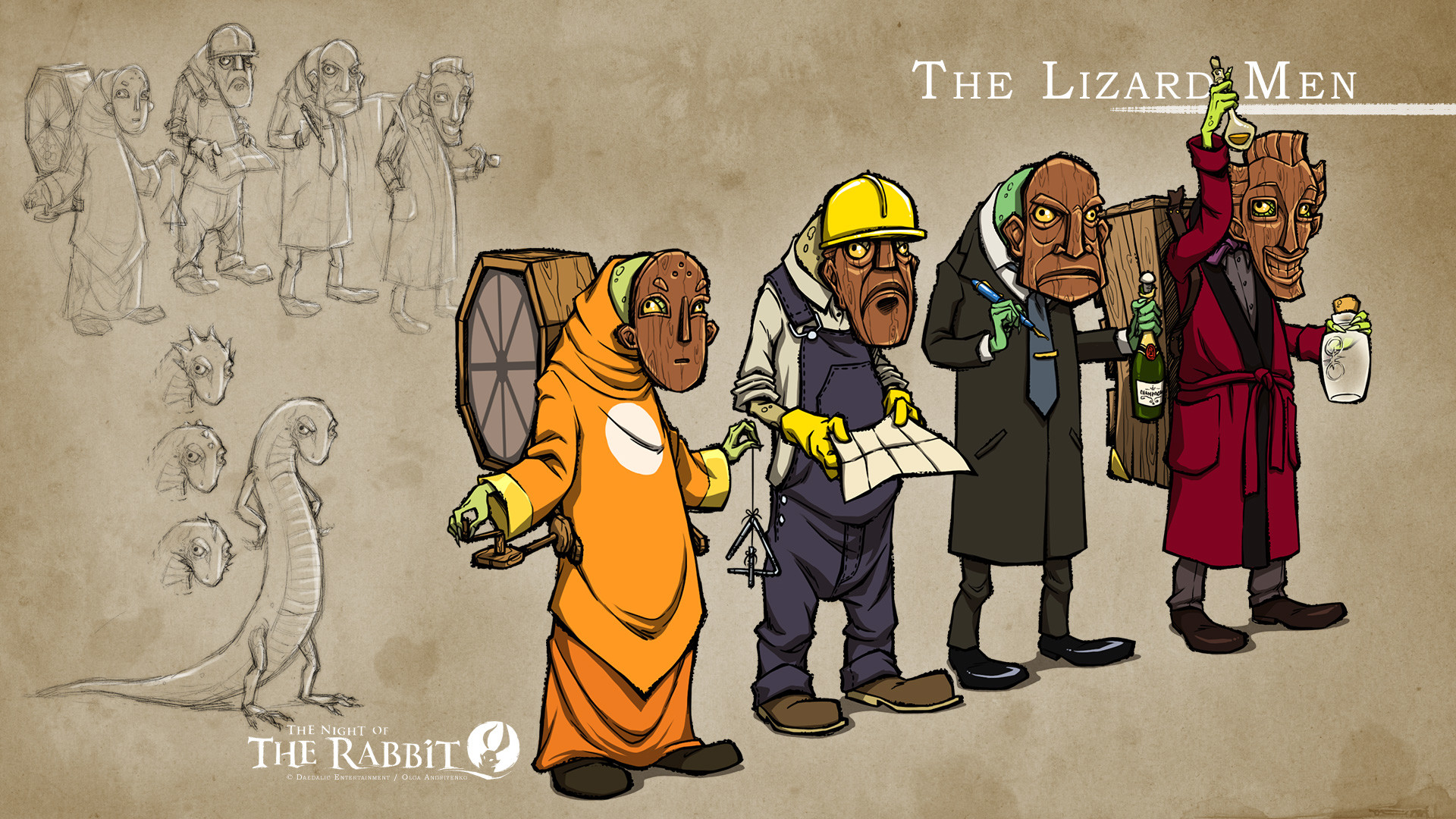The image is a horizontal rectangular cartoon-style illustration with a light brownish-gray, diffused background. The left-hand side of the image features detailed pencil and chiaroscuro sketches of characters and a standing lizard with its hands on its hips. Below these are three differently-expressed lizard heads, and the text "The Knight of the Rabbit" is visible. On the right-hand side, taking up about two-thirds of the image, are the fully-colored and developed cartoon characters labeled "The Lizardmen" in the top right corner. The four lizard characters, all cunningly disguised in various human outfits, range from a businessman in a suit and tie, a construction worker with a yellow hard hat, to one in a maroon dressing gown holding a bottle, and another in an orange robe with a wooden object on his back. The lizards wear brown face masks made of wood, blending their reptilian features with their human attire.